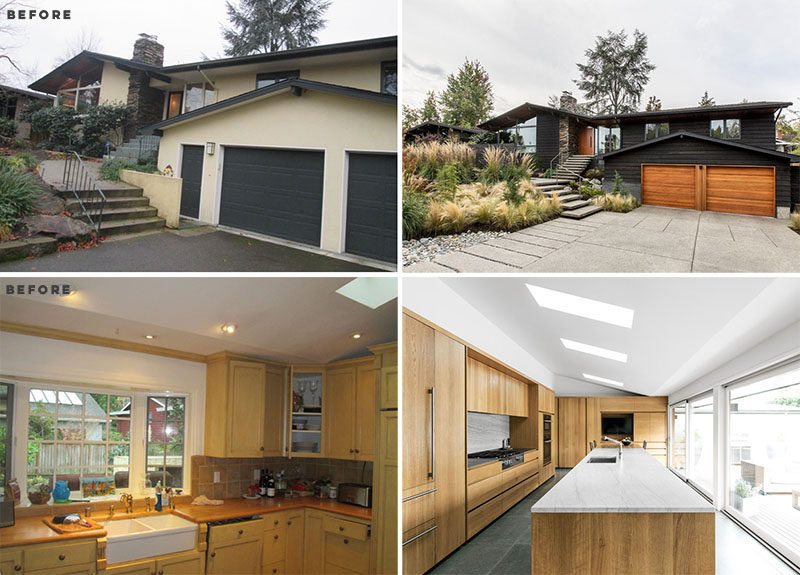The image showcases two sets of "before and after" photographs detailing the extensive renovation of a house and its kitchen. In the top-left quadrant, an initial view of the house highlights light cream-colored walls, a black roof, a prominent black garage door framed in white, and a rock-shaped chimney with a green tree in the background. A concrete stairway with a metal railing ascends to the left side of the house. Next to this, the after renovation photograph reveals the house transformed with sleek black walls and wooden paneled garage doors in a light brown hue.

The bottom left corner presents the pre-renovation kitchen, characterized by yellow-colored cabinets, a white recessed sink, and a large window with approximately ten individual panels. The adjacent post-renovation view depicts a modernized kitchen featuring a sloped ceiling with three square lights, a central island topped with light gray granite, and a black, wall-integrated stovetop on the left. New, large two-panel windows replace the older style, inviting ample natural light into the revamped space.